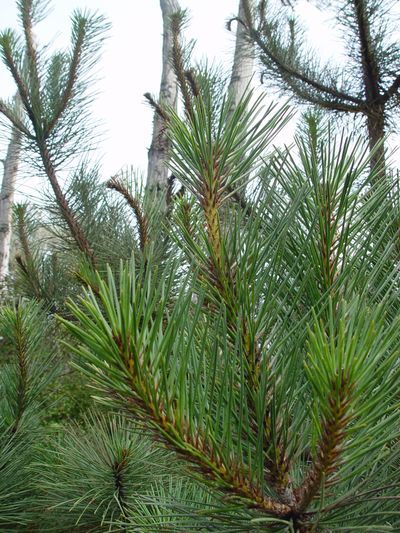This image is a detailed, up-close photograph of a pine tree taken outdoors during the daytime. It captures a zoomed-in view of a pine branch, prominently displayed in the bottom right-hand corner of the photo. The branch has a distinctive W shape and showcases the tiny green spikes that form the needles of the tree, which appear sharp and pointy. The needles transition from light green at the tips to a darker green closer to the center of the branch, giving the branch a full and lush appearance reminiscent of a real Christmas tree. The limbs of the branch exhibit some brown coloration. In the background, several tree trunks without leaves, possibly from birch or other leafless trees, rise into view, adding contrast to the vibrant green of the pine needles. The perspective of the photograph appears to be from ground level, looking up at the tree.